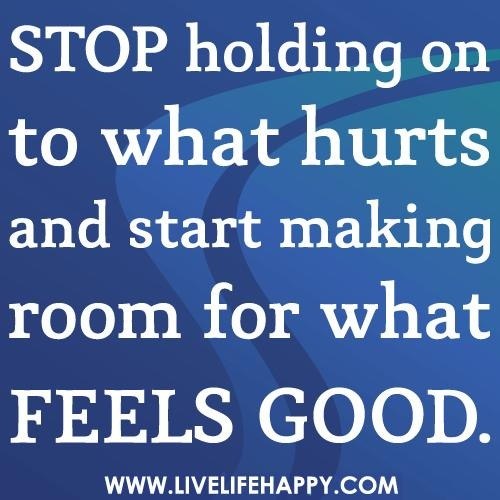The image is a blue square featuring an intricate design with lighter blue elements. White text boldly fills the width and height of the square with the phrase: "STOP HOLDING ON TO WHAT HURTS AND START MAKING ROOM FOR WHAT FEELS GOOD." Notably, "STOP" and "FEELS GOOD" are in all caps to emphasize their importance. Below this text, "WWW.LIVELIFEHAPPY.COM" is also in all caps, serving as a footer to the message. The background includes a thin squiggly curve on the left and a large oval-shaped darker blue section on the right, consisting of three layered wave patterns. The font includes subtle serifs, and the "A" displays a slightly fancy design, giving a touch of elegance to the otherwise simple script.